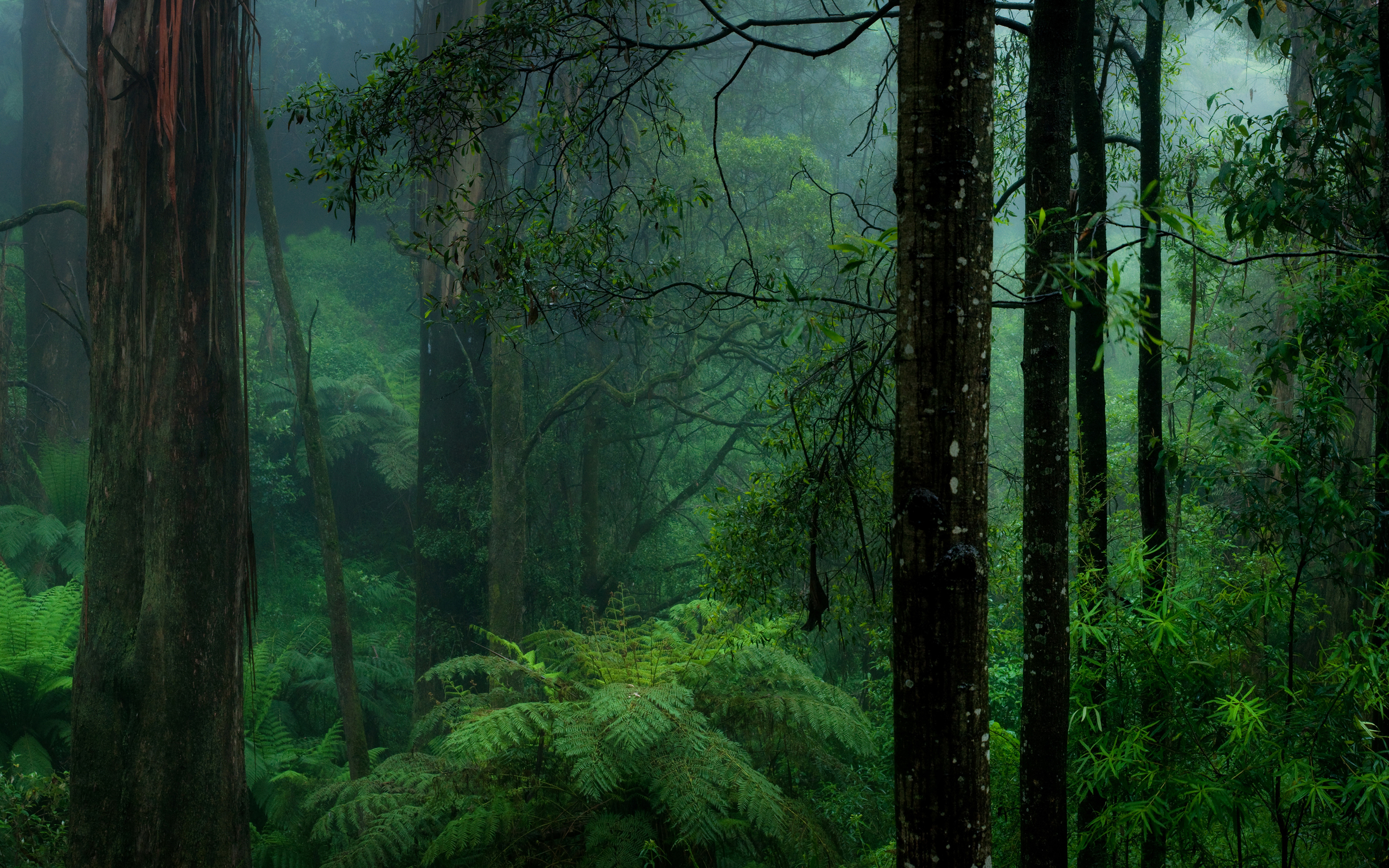The painting portrays a dense, overgrown jungle scene, rich in greenery and various textures. Dark and misty, the forest gives an impression of dawn or dusk, with little to no sunlight penetrating the canopy. On the left side, a prominent tree with a thick trunk stands, adorned with wooden-like vines that cascade downward. To the right, several slender trees are visible, their trunks covered in moss, contributing to the forest's damp, untouched ambiance. The forest floor is lush and diverse, featuring tall grasses, expansive ferns, and an array of dense green plants in various shades from dark to light green. Overhanging branches create a canopy that shadows the forest floor, adding to the scene’s mysterious and timeless feel. In the top right corner, a subtle light filters through the treetops, casting a grayish tone over the middle of the forest. The terrain appears to slightly rise towards a hill, beyond which distant mountains peek through the mist. The overall atmosphere is one of raw, unspoiled nature, where the dense vegetation and foggy air suggest a land untraversed by humans.